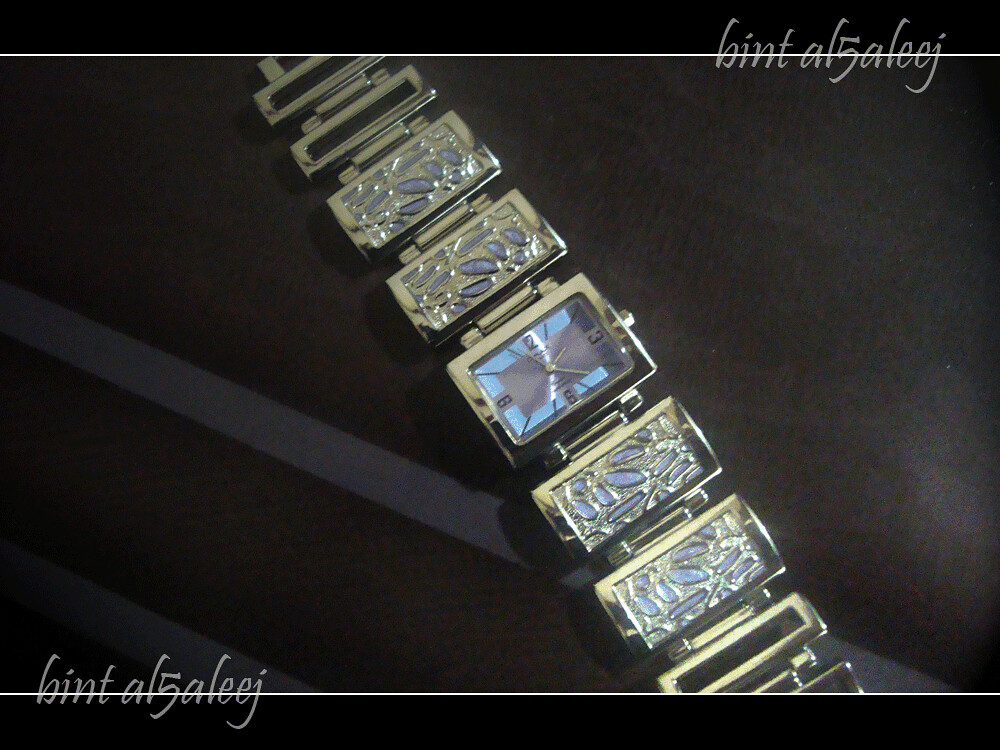This is a detailed descriptive caption for the provided image of a watch face:

"The watch face is rectangular and framed with a sleek steel bezel. The background is black, accentuating the prominent white markers positioned at 12, 3, 6, and 9 o'clock. Additional smaller hour markers fill in the intervals. At the bottom of the display, there is a partial signature, with visible sections at both the bottom left and the top right corners. The date display is presumably located on the watch face as well, although its exact position isn't specified. A hint of the numerals 'l5 a l e e j' is subtly etched at the bottom of the watch face."